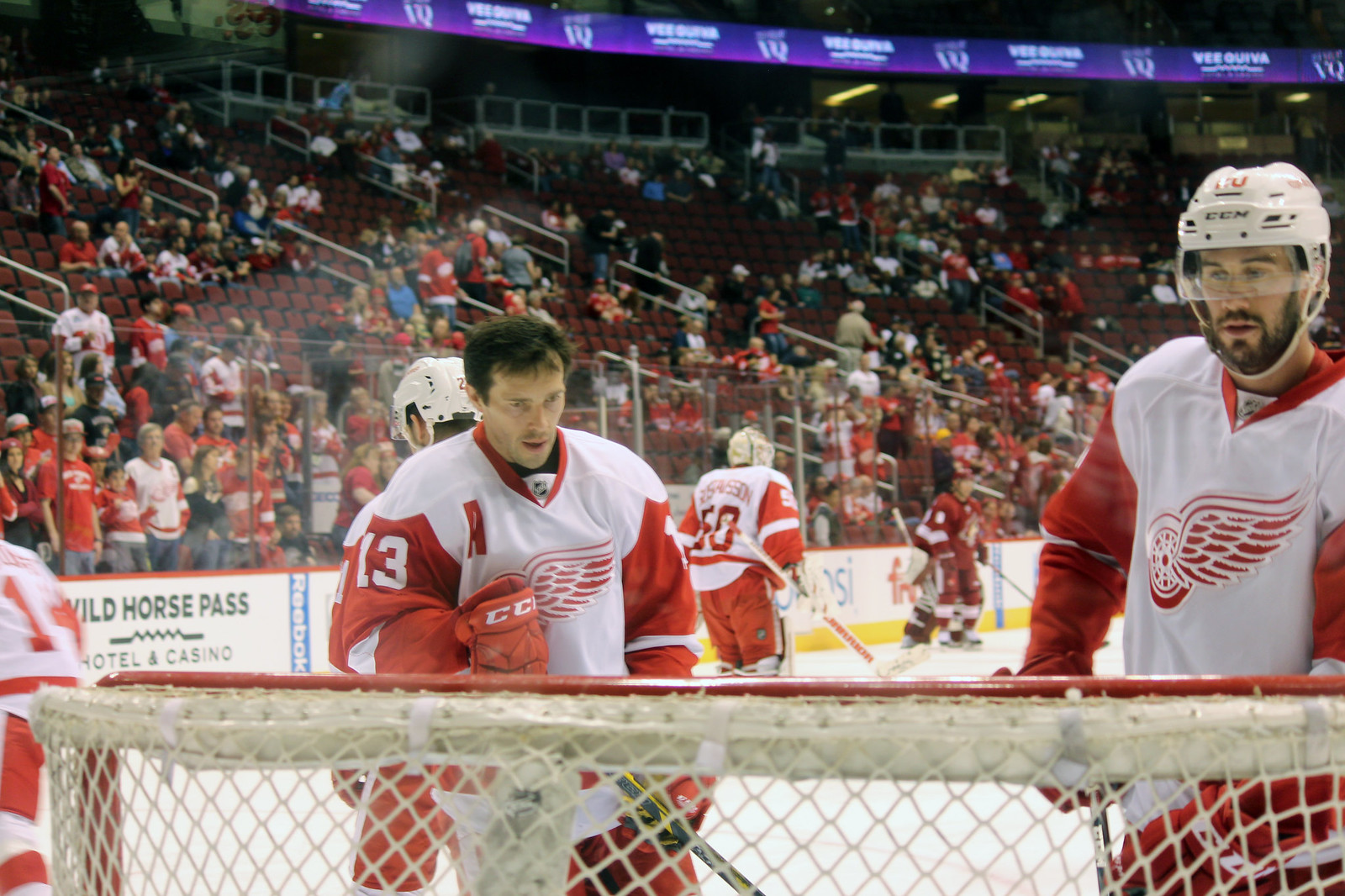This photograph captures an intense and dynamic moment from a Detroit Red Wings hockey game. Taken from a wide, rectangular perspective behind the goal, the image prominently features the net with its red metal border and white mesh. Two main players are in focus, one tall player donned in a white helmet, white jersey with red sleeves, and red gloves, is positioned to the right, gazing down towards the goal. The distinct Red Wings logo, a red and white winged wheel, is prominently displayed on his chest. To the left, slightly off-center, a shorter player without a helmet can be seen, also wearing the same uniform, with the number 13 visible on his left shoulder. Both players appear to be taking a brief respite, looking away from the rink, indicating a pause in the game. The stands behind them are packed with fans, many dressed in red, reflecting the local support and creating a vibrant atmosphere. The spectators in the front rows are on their feet, suggesting a recent intense moment or a significant play. Visible sponsor advertisements like Reebok and Wild Horse Pass Hotel and Casino are displayed on the rink's side paneling, adding to the authentic feel of this large indoor arena.